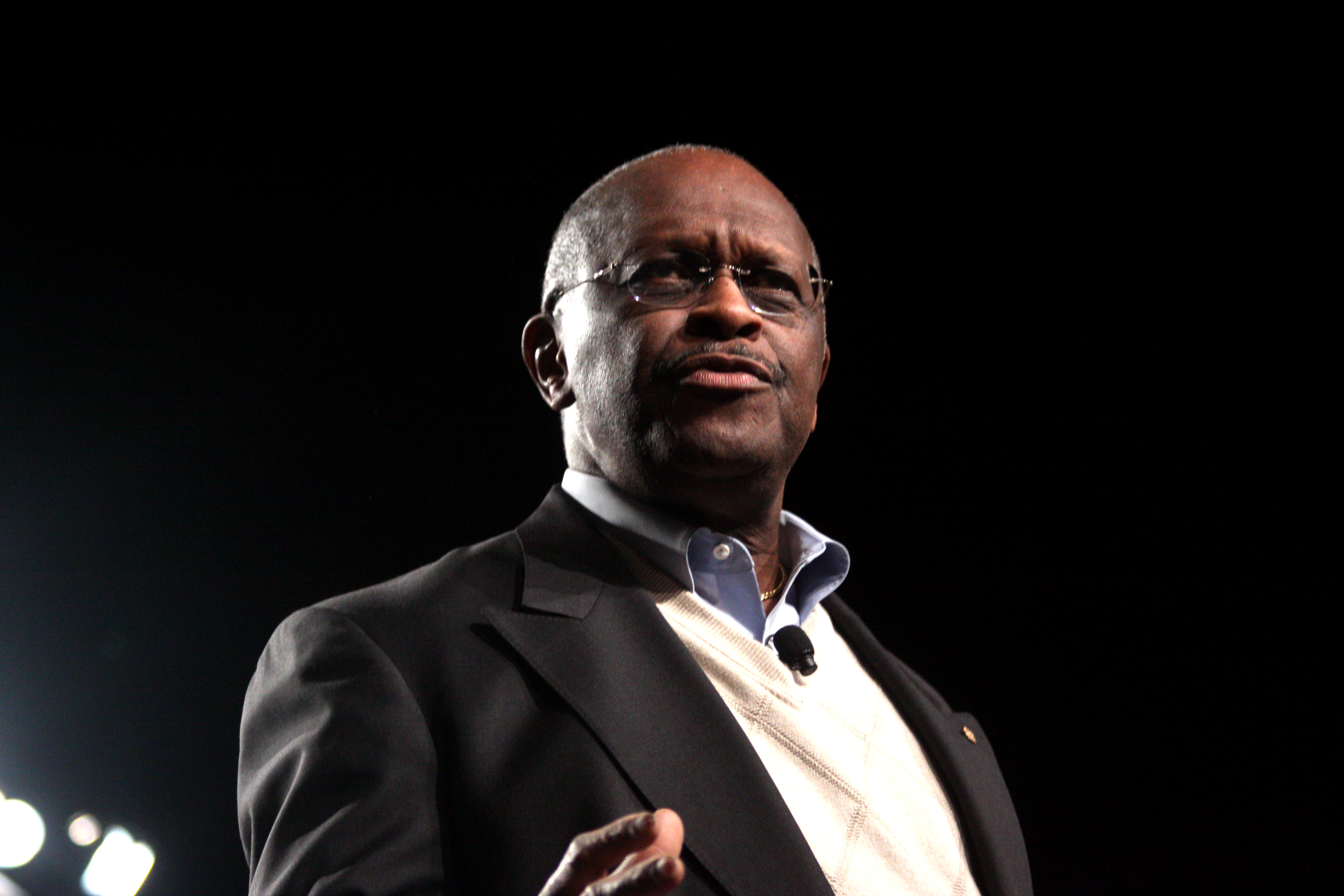The image captures a distinguished black male, who appears to be giving a speech amidst a dark, nighttime background. He is clad in a black suit jacket adorned with a gold pin on the chest and a white V-neck sweater layered over a light blue button-down collared shirt, unbuttoned at the top. A small black microphone is attached to his sweater, and a delicate gold necklace peeks out from beneath his layers of clothing. The man, an older individual with short grayish hair and a black pencil mustache, also wears clear oval glasses. He is gesturing with one hand as he speaks. Notably, this man was a politician, famously linked with a "999" slogan, who ran for presidency on the Republican side, possibly against Trump, and passed away due to COVID-19. The image includes illumination from a spotlight in the lower left-hand corner, casting light on his figure amidst the otherwise black, sky-like background.